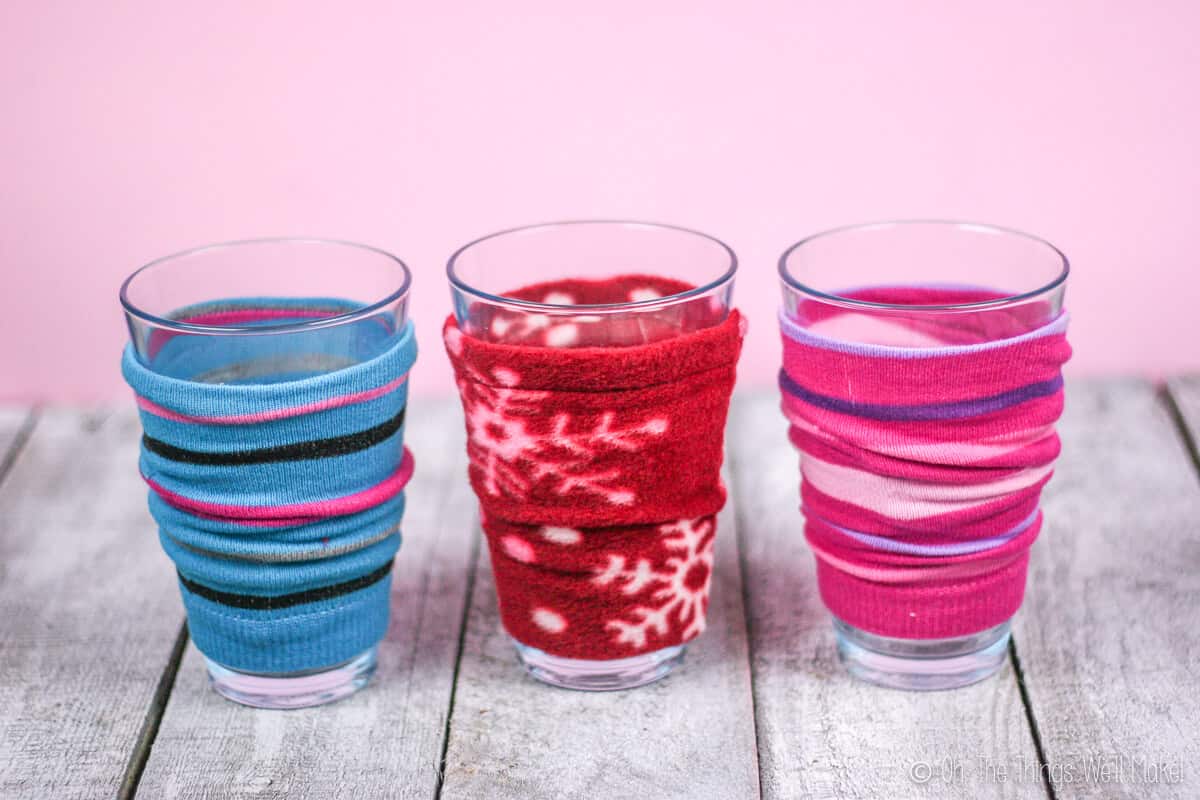In the image, three simple clear water tumblers are centered on a rustic, gray wooden surface resembling a table or deck. Each tumbler is adorned with a distinctive elastic fabric wrap, akin to a cozy, likely to prevent condensation. The backdrop is a light pink wall. The first tumbler features a wrap with blue, turquoise or purple, and black stripes. The middle tumbler sports a red fleece wrap embellished with white snowflakes and dots, evoking a holiday theme. The third tumbler is wrapped in a pink fabric with purple and lavender stripes, along with a possible white stripe in the middle. The wooden surface's light, palette-like appearance contrasts subtly with the colorful, cozy-clad glasses and the soft pink background.